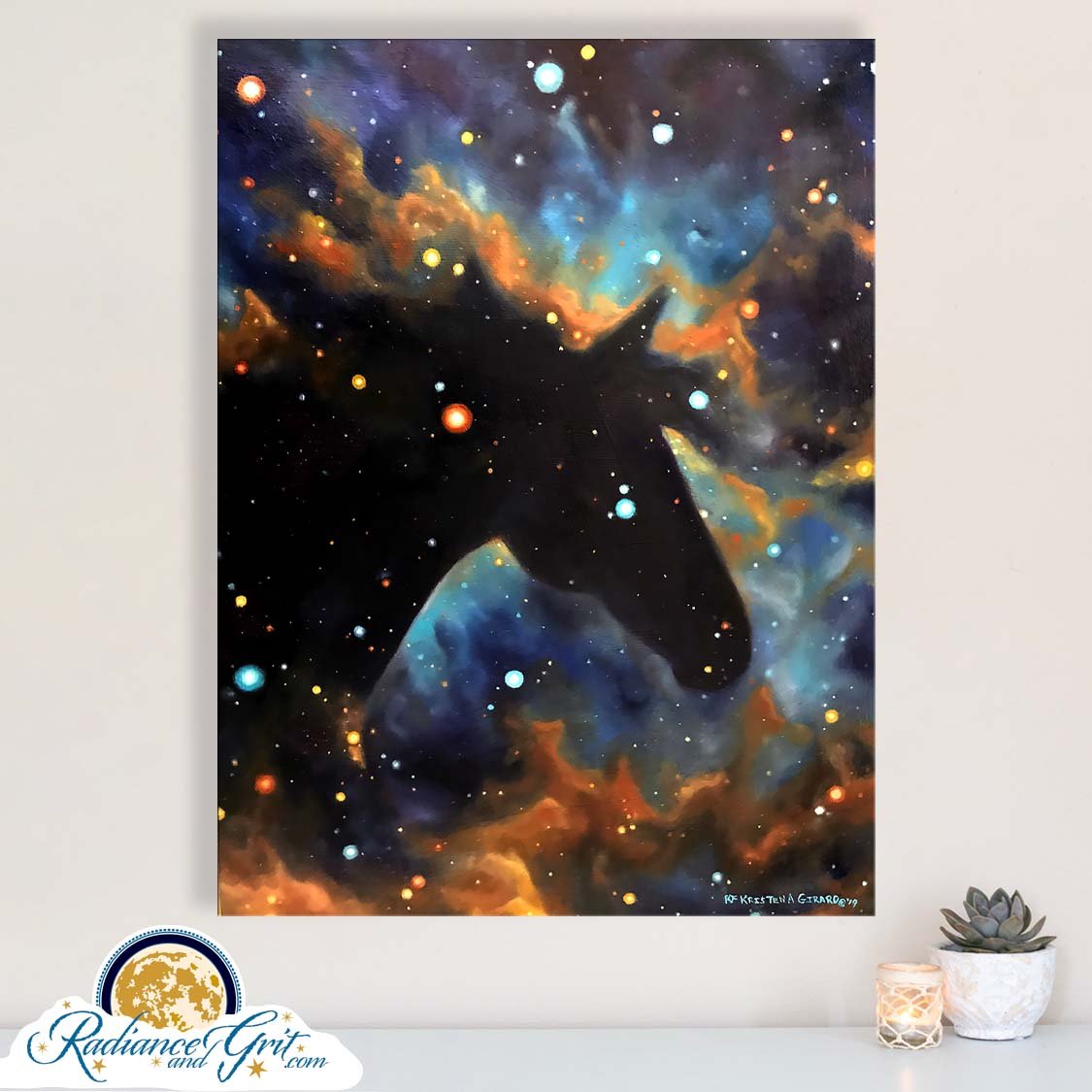This image depicts a framed poster elegantly fixed on a light beige wall. The artwork itself is a mesmerizing digital or spray-painted representation of a galaxy or nebula, featuring a shadowy silhouette of a horse at its center. The cosmic scene is composed of deep black and darker blue hues, accented with scattered dots of light blue, orange, yellow, red, and white, depicting stars of various sizes. Below the poster, on a shelf to the bottom right, sits a low-burning candle beside a small white pot holding a succulent. Off to the left beneath the poster, a cursive dark blue to teal font spells out "Radianceandgrit.com," indicating the probable source or seller of this art piece. The overall composition suggests an advertisement, enhanced by the enigmatic figure of the horse set against the celestial backdrop.